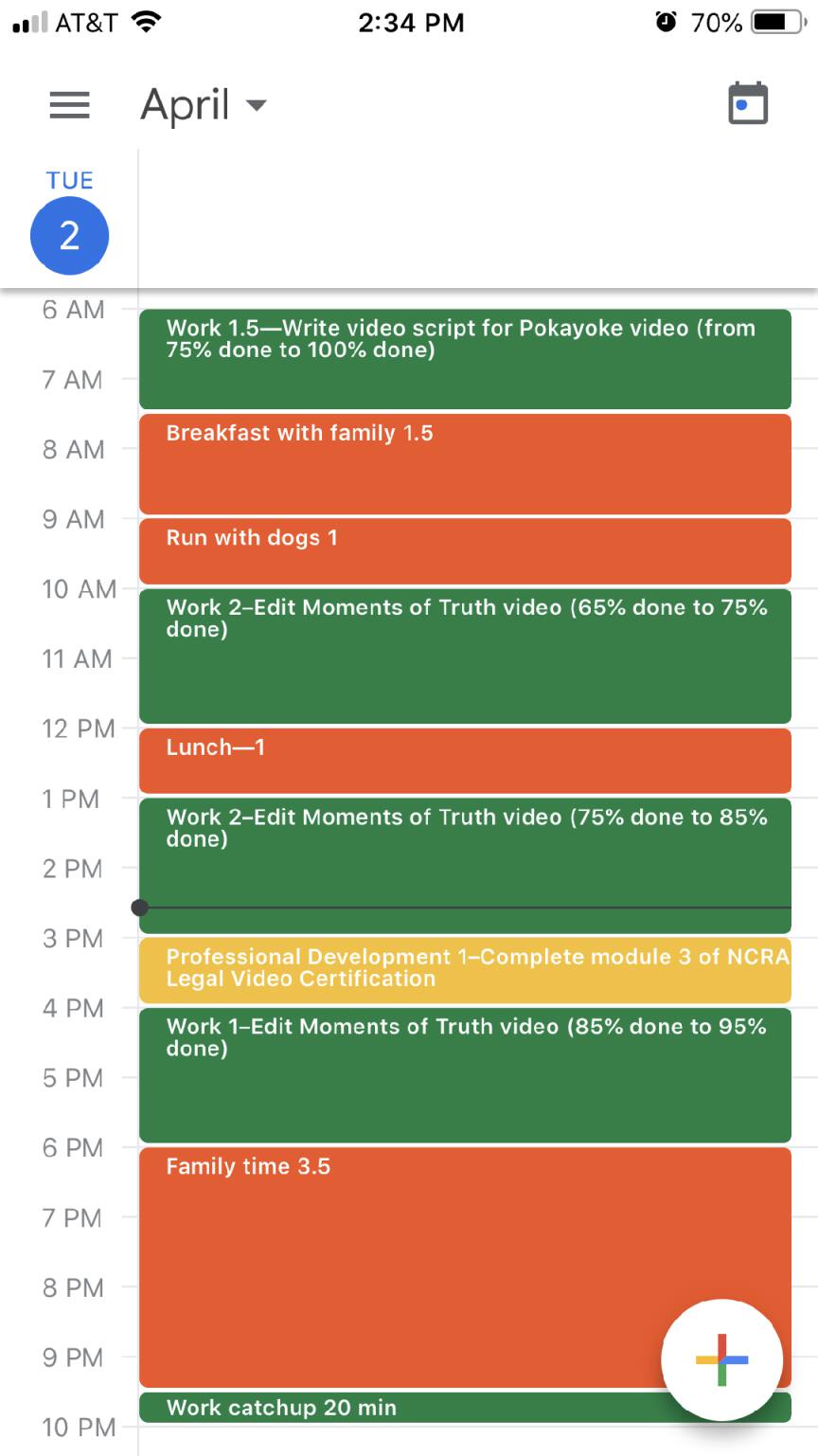A detailed portrait of an iPhone screen displays various elements indicating its status and functionality. In the top-left corner, the signal strength meter shows two out of four bars in black, signifying an AT&T connection with moderate signal strength. Next to it, the fully lit Wi-Fi symbol signifies a strong wireless connection. The current time is displayed as 2:34 p.m., adjacent to an illuminated alarm clock icon. The battery indicator, positioned at the top right, shows a 70% charge level in a horizontal format.

Below these status indicators, the screen showcases an app interface. In the top-left corner of the app, three horizontal lines represent a menu icon. To the right, the word "April" is displayed with a down arrow, suggesting a dropdown menu for selecting different months. Further right, there is a calendar icon featuring a blue dot near the upper left corner, indicating an event or reminder.

Underneath this, the abbreviation "TUE" (Tuesday) is shown prominently along with the date "2" in white, set against a blue circular background. The left-hand column of the screen enumerates time slots from 6 a.m. to 10 p.m. in one-hour increments. To the right of these time markers, various event cards are displayed, each marked with white text. These cards have backgrounds in various shades of green, orange, and yellow, indicating different categories or statuses of events.

In the lower right corner, a plus icon commonly used by Google is encircled in white, suggesting an option to add new entries or events to the schedule.